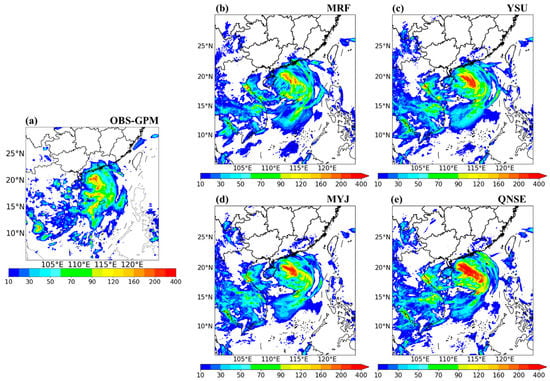The image comprises five radar panels that together illustrate the progression of a storm moving from the southwest to the northeast over a designated land area. Each panel features a color-coded bar beneath it, detailing the intensity levels of precipitation: dark blue and light blue signify clouds and light rain, green indicates moderate precipitation, yellow shows a higher degree of precipitation, and red represents the highest precipitation levels and potential lightning activity. The five panels are arranged with one on the left and four stacked in a two-by-two grid on the right. Latitudinal and longitudinal degrees are marked on the left side of each panel, providing geographical context. The labels OBS, GPM over 1, MRF, YSU, MYJ, and QNSE are displayed on the image, possibly indicating different tracking or weather models used in the analysis. Three of the panels prominently show areas marked in red, denoting intense storm conditions.